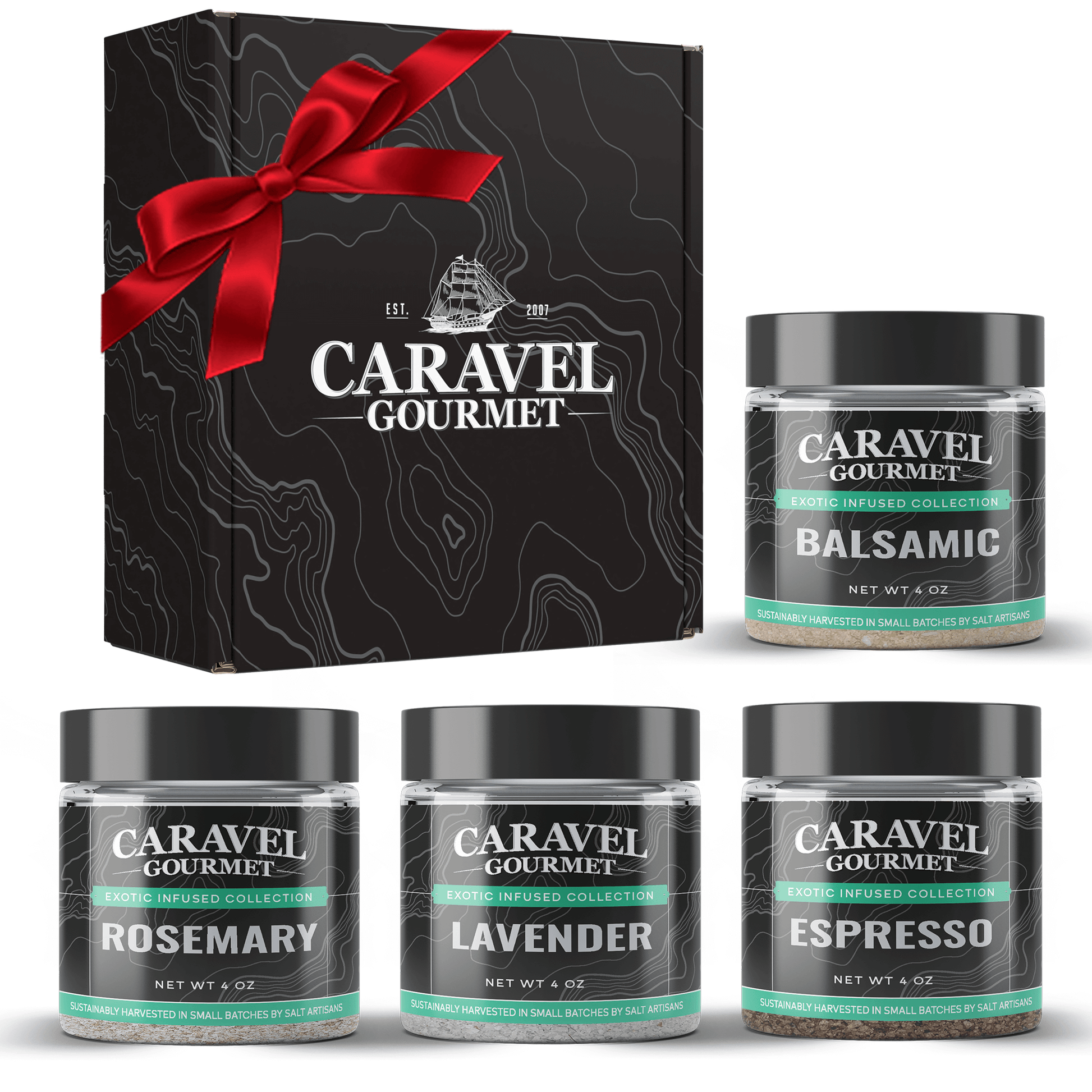The image depicts a gift box labeled "Caravel Gourmet" with a distinctive red bow tie, situated in the top left corner. The black gift box, adorned with a white line pattern reminiscent of a geode texture, houses four small spice containers. Each bottle is marked with the Caravel Gourmet logo featuring an old-fashioned sailing ship and the inscription "EST 2007." The spice containers, each with a black lid and green label, are part of the "Exotic Infused Collection," sustainably harvested in small batches by salt artisans. The flavors included in this set are balsamic, rosemary, lavender, and espresso, and each bottle has a net weight of four ounces. The visually appealing labels, with clear white font on a black background, make the set look like an attractive offering from a catalog or a website where it can be purchased.